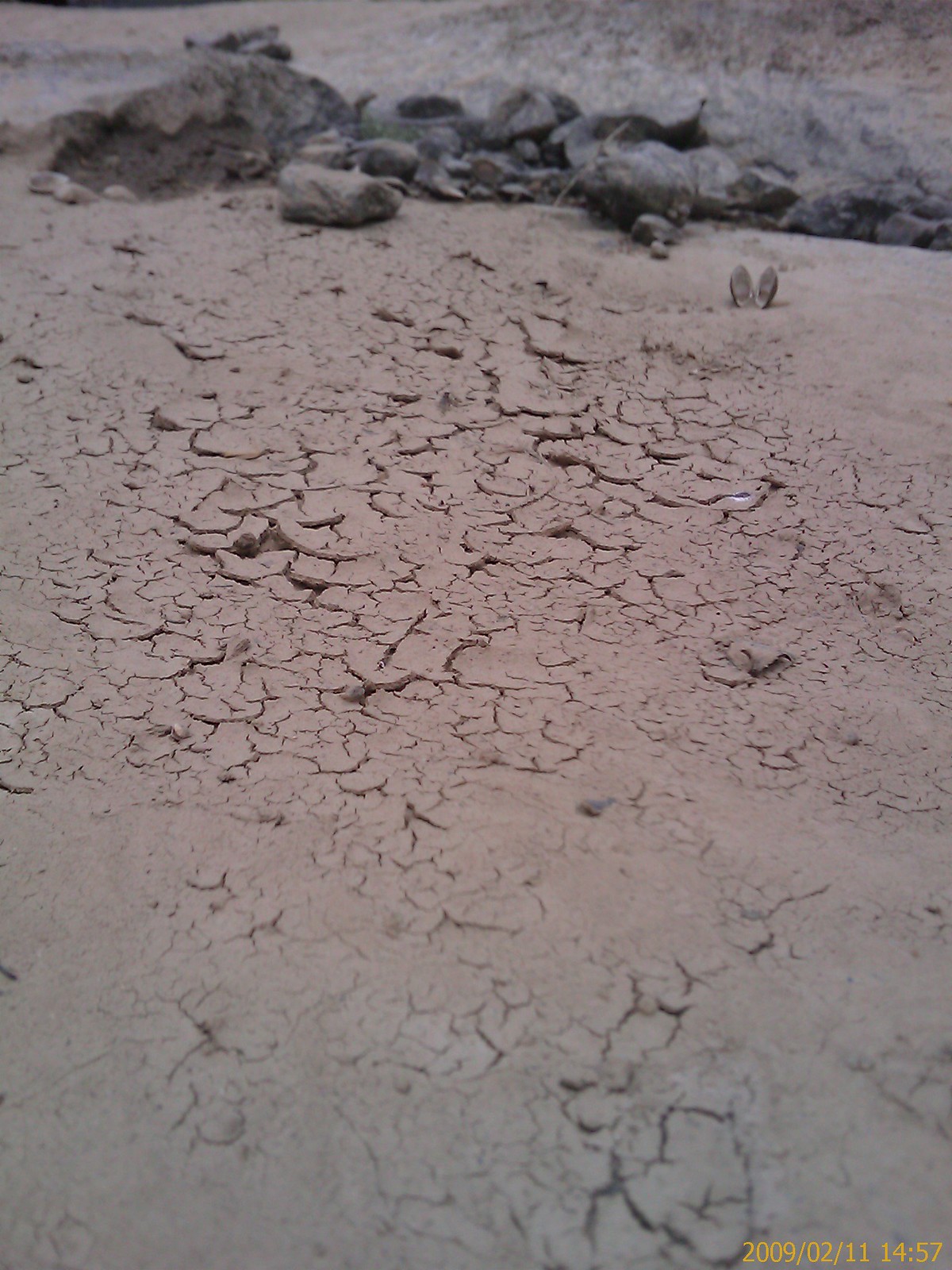The photograph, captured in portrait orientation, displays a desolate, arid landscape characterized by dry, cracked, and flaky ground reminiscent of dried mud or clay, with hues of brown, gray, and subtle orange and pink undertones. The surface appears old and corroded, resembling the way skin dries and flakes. At the top of the frame, a collection of dark gray, dirt-covered rocks punctuates the barren scene, further emphasizing the lack of vegetation throughout the image. The bottom right corner features a yellow timestamp from the camera, dated 2009/02/11 at 14:57.